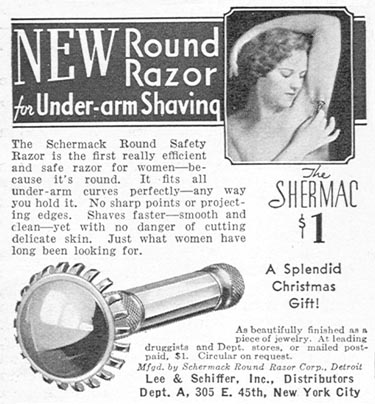This image is a black-and-white advertisement, likely from a magazine or newspaper, promoting the innovative Shermack Round Safety Razor for underarm shaving. In the top right corner, there is a woman with short permed hair demonstrating the use of the razor by shaving her left underarm with her right hand. The text prominently highlights the benefits of the razor, stating that it is the first truly efficient and safe razor for women. Its round design fits all underarm curves perfectly, no matter how it is held, and it features no sharp points or projecting edges, ensuring a fast, smooth, and clean shave without the danger of cutting delicate skin. Below this, a detailed drawing of the razor is shown in the lower left corner, accentuating its unique, jewelry-like finish. The caption describes the razor as an excellent Christmas gift available for $1 at leading druggists and department stores or via mail post-paid. The manufacturer is Shermack Round Razor Corporation, Detroit, with distribution by Leon Schiffer Inc., Department A, 305 East 45th, New York City.